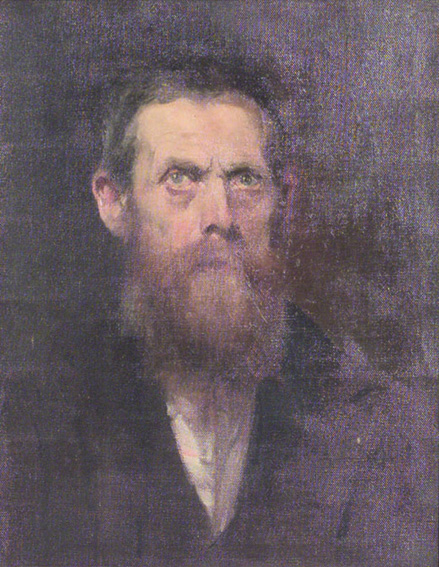The artwork is an oil painting of a white middle-aged man, portraying a highly detailed, somber portrait. His face exhibits signs of aging with lines on his forehead, bags under his blue eyes, and a somewhat unkempt appearance, characterized by a straggly brown beard and mustache, and receding hairline. The man is dressed in a dark brown jacket that nearly blends into the grayish-black background, adding a muted, monochromatic tone to the piece, with his white shirt providing a stark contrast. His complexion has touches of rose, particularly on his cheeks and ears, with his right ear appearing notably large and red. The man gazes slightly upward, not directly at the viewer, imparting a sense of introspection or focus on something above him. The overall dark tones and subtle use of color accentuate the stern, contemplative expression on his face, making it an intriguing and thoughtful portrait.